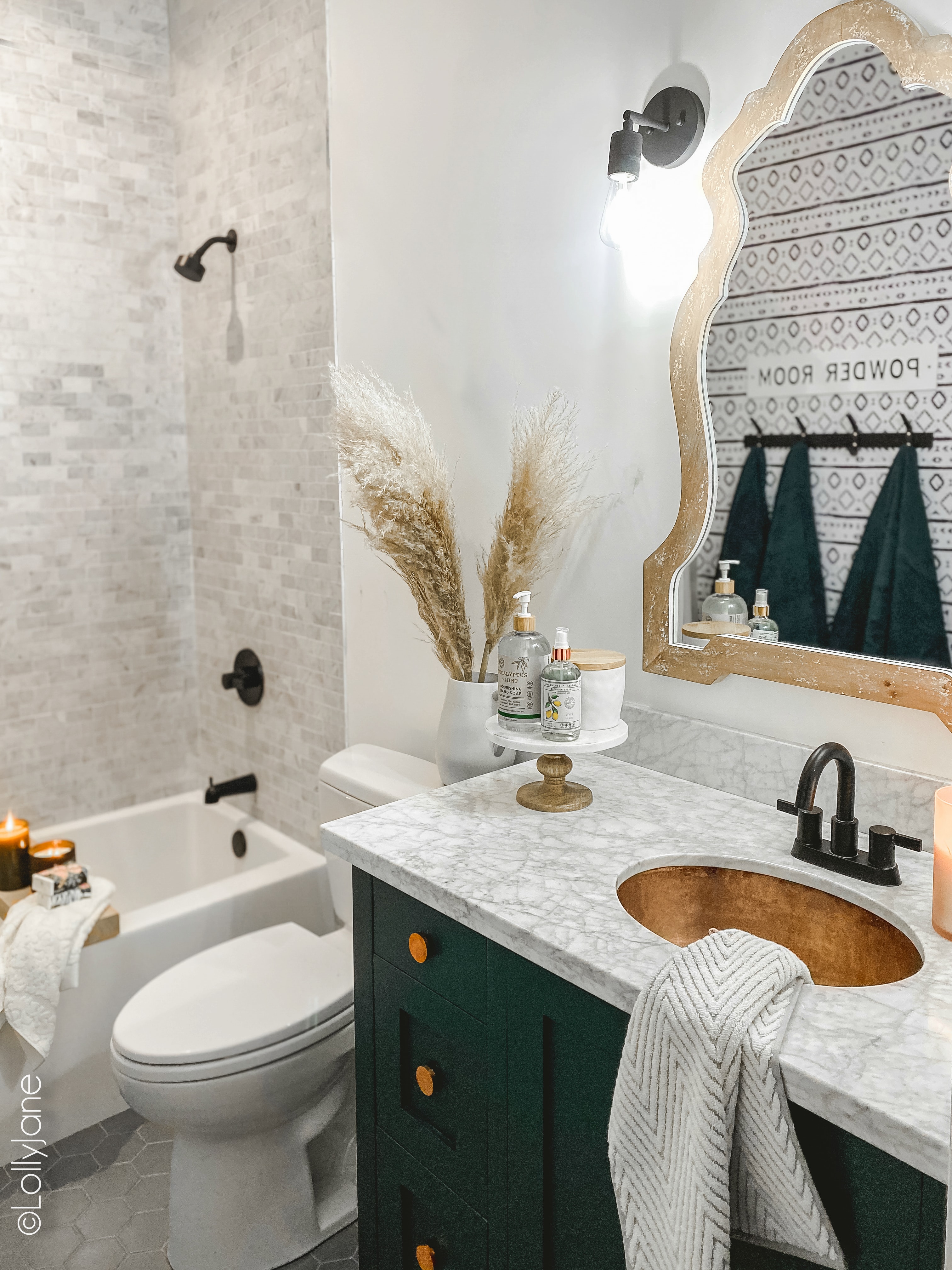This detailed rectangular image captures a luxurious home bathroom. The overall color scheme is white and pale gray, creating an elegant ambiance. On the left side, there is a stylish shower area adorned with grayish stone-like tiles and sophisticated black fixtures. A bathtub is located nearby, featuring a bath tray that holds lit candles, soap, a towel, and other small items, suggesting a relaxing atmosphere.

In the center of the image, a white toilet sits between the sink and the bathtub. Above the toilet, there's a white ceramic vase containing beautiful dried fronds in brown and white, adding a touch of natural decor.

To the right forefront, a small sink with a stunning white and gray marble countertop stands out. This sink is equipped with a sleek dark bronze faucet. Above the sink hangs an elegantly curved mirror in a pale gold frame, reflecting a black towel rack adorned with dark blue towels. The word "Powder Room" is noticeable on the wallpaper, further enhancing the room's sophistication. The basin area also includes soaps, a gray and white towel, and candles, enhancing the overall aesthetic of this finely detailed bathroom.